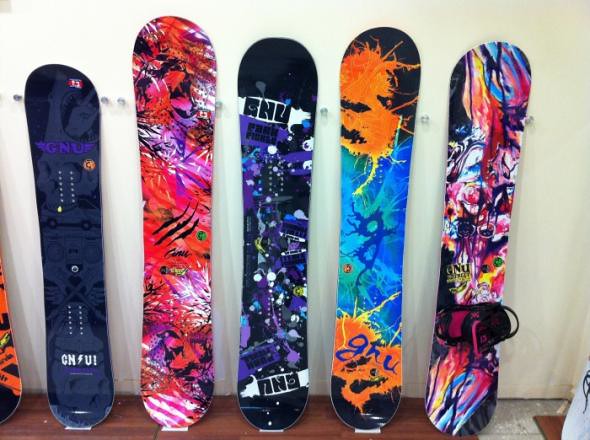The photograph showcases five vibrant, multicolored snowboards leaning vertically against a wall. They are secured by small pegs or clasps on the wall, ensuring they remain upright and displayed prominently. Starting from the left, the first snowboard features a dynamic blend of black, blue, and purple hues. The second snowboard stands out with its striking combination of red, black, white, and pink, adorned with floral patterns. The third snowboard has a captivating mix of black, purple, and green, with highlights of blue. The fourth snowboard primarily exhibits a bright blue center with intricate designs and black ends with orange accents. The fifth and final snowboard is an explosion of colors including red, pink, white, yellow, and green, and it includes a visible bootstrap for securing boots. Additionally, there is a glimpse of an orange snowboard with brown or blue edges just slightly visible behind the others. The snowboards rest on a wooden surface, and their varying heights suggest an array of styles and purposes.